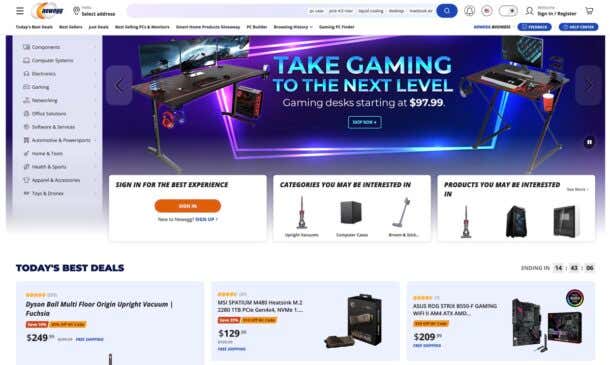This image depicts a website's homepage, viewed from left to right in a horizontal layout. The background of the website alternates between white and its own distinct design elements. 

At the top-left corner, there are three horizontal lines representing a menu for additional options, followed by a slightly blurry company logo. Moving towards the center, a search bar is prominently displayed. To the right of the search bar, there are various icons including a magnifying glass indicating the search function, a bell for notifications, a profile icon, and a shopping cart icon positioned at the far right. Adjacent to the shopping cart icon is the sign-in/register button. 

Beneath the top navigation bar, the background turns white with some clickable options in black, though they appear blurry. Continuing to the right on the same row, several clickable options in blue are visible.

On the left-hand side of the main content area, a periwinkle-colored sidebar is present, featuring different categories and tabs in black text for user navigation. 

To the right of this sidebar, a featured banner with a dynamic purple and iridescent blue background is showcasing a promotion: "Take Gaming to the Next Level." This banner includes an image of a gaming desk with the text "Gaming desks starting at $97.99." There are images of two desks flanking the promotional text.

At the bottom of the image, a section labeled "Today's Best Deals" highlights various products on sale, continuing the theme of the homepage.